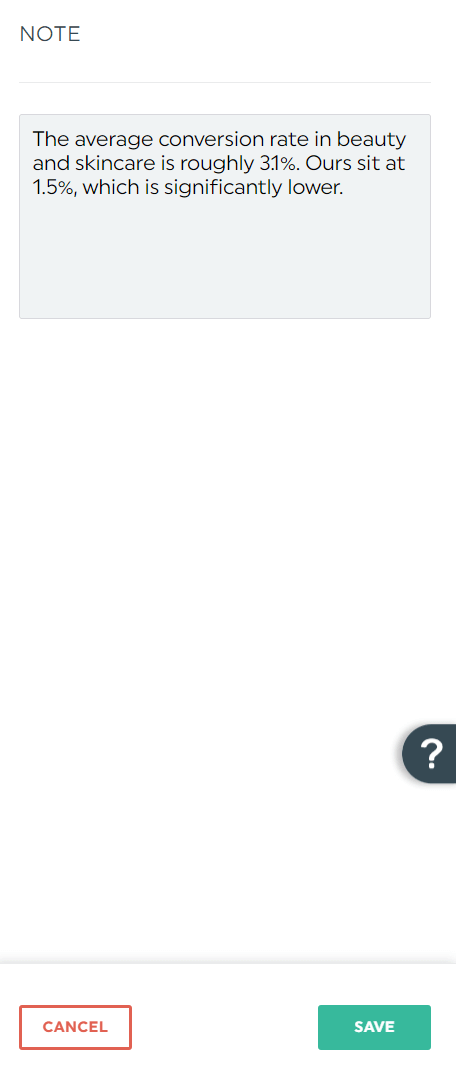The background of the image is white. In the top left corner, there is the word "NOTE" written in all capital letters in gray, followed by a thin gray line that extends horizontally across the width of the image. Below this line is a gray rectangle with the words "The Average Conversion Rate and Purity" written in dark gray, with "The" capitalized.

The next line within the rectangle reads, "ASN care is roughly 3.1%," followed by a period. The subsequent line states, "Ours sit at 1.5%," followed by a percent sign and a comma, and continues with, "which is significantly lower," ending with a period. The remaining space within the rectangle is blank.

As you move further down the image, the background remains white. There is a gray semi-circle (or semi-oval) with a white question mark inside it. Continuing downward, another thin gray line extends across the width of the image.

Below this line are two buttons. The first button has a white interior with a red border, and the word "CANCEL" is displayed in bold red capital letters. The second button has a green interior with the word "SAVE" written in bold white capital letters.